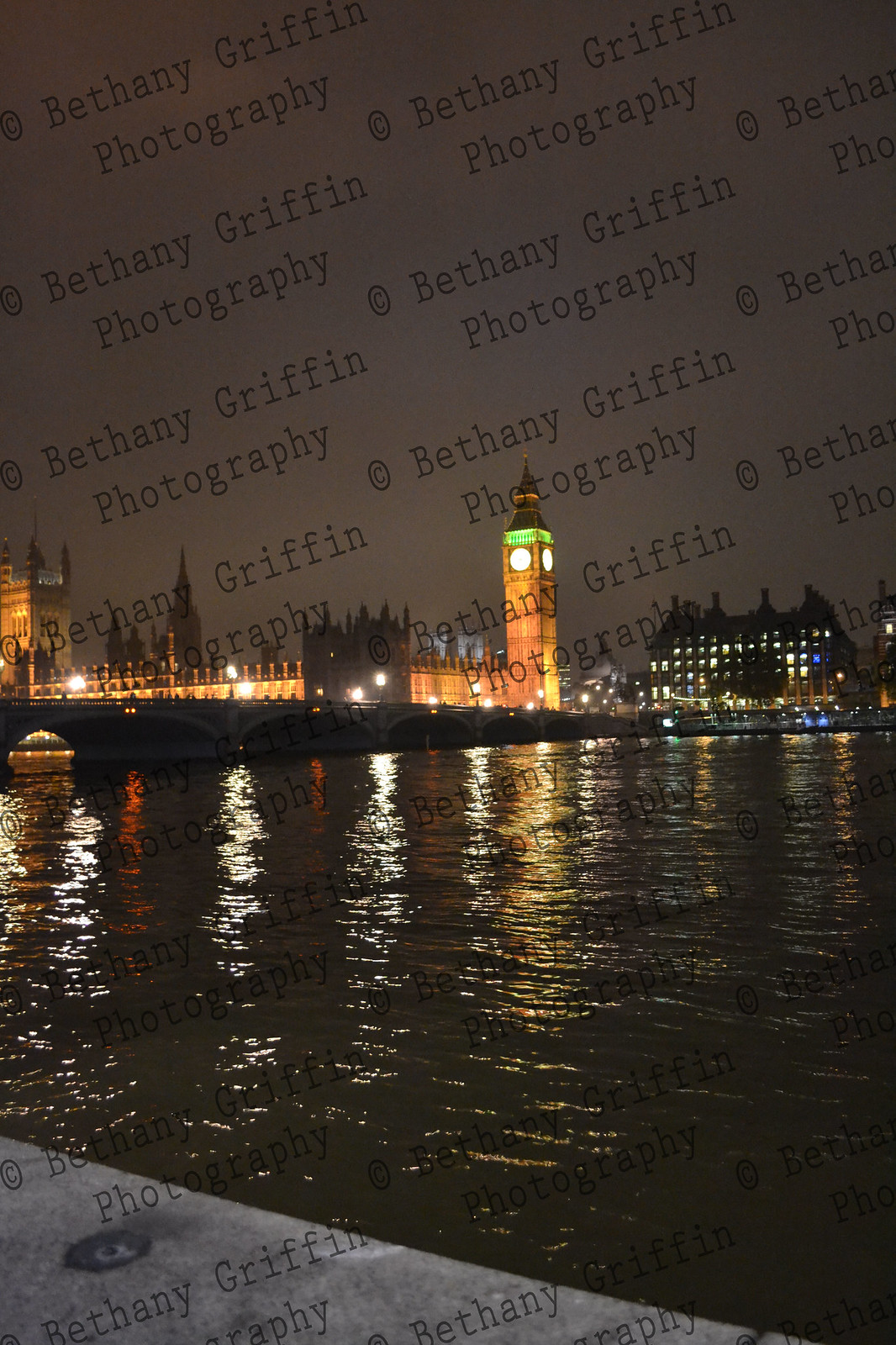This nighttime photograph captures a vibrant cityscape dominated by a large, illuminated clock tower displaying time on two visible sides. The clock tower stands amidst an array of buildings that vary in height, with many featuring pointed, triangular roofs piercing the dark, grayish night sky. Some buildings are illuminated with glowing windows, while others remain dark. A prominent bridge stretches from left to right, leading towards the city, adding a sense of connection and depth to the scene.

In the foreground, a vast body of water—possibly a port, river, or pond—reflects the city lights, creating a mirror-like effect. The water spans nearly half of the image, separating the photographer's vantage point from the distant cityscape. Close to the edge of the water, a concrete promenade where people might stand and gaze over the scene is barely visible.

This scene unfolds under the watermark of 'Bethany Griffin Photography,' repetitively printed across the image, providing a subtle yet somewhat distracting layer to the overall composition. The photograph not only highlights the city's architectural elegance with its well-lit structures and majestic bridge but also captures the serene expanse of water under the night sky.